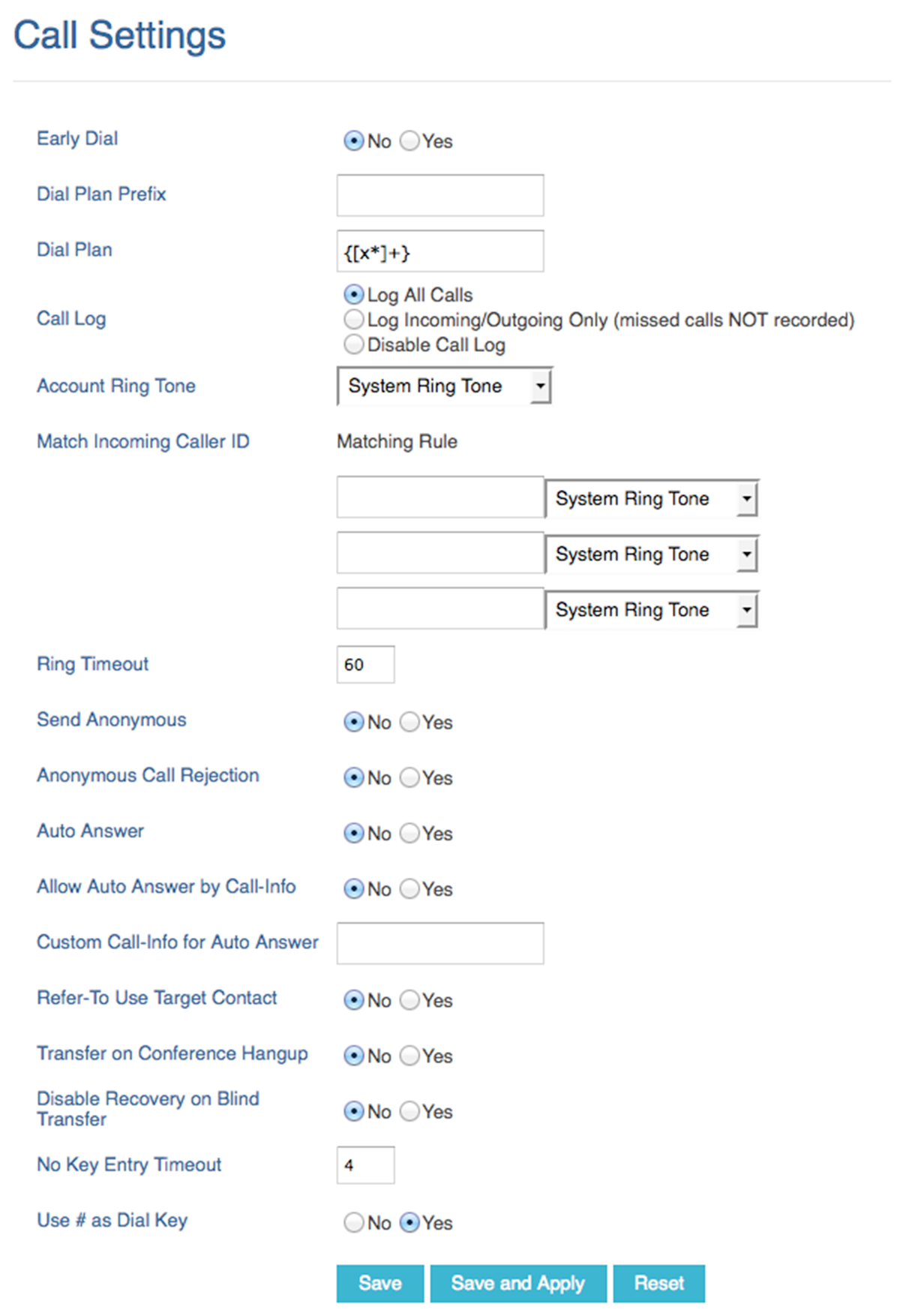### Detailed Screenshot Caption

The screenshot displays a web page containing a settings interface with various configurable options. At the top of the page, there is a header with a broad, horizontally-aligned blue title text. Directly below this title, a dividing line segregates the header from the rest of the settings interface.

The settings are organized into distinct sections to the left, each identified by blue text, and corresponding input fields or options to the right. The sections are as follows:

1. **Early Dial**: This section offers two radio buttons labeled "No" and "Yes" to select between disabling or enabling early dialing.
2. **Dial Plan Prefix**: An empty field is provided where users can input a prefix for their dial plan.
3. **Dial Plan**: This section includes a field containing a pre-filled formula for the dial plan.
4. **Call Log**: Users can choose between three vertically stacked radio buttons: "Log all calls," "Log incoming/outgoing only," and "Disable call log."
5. **Account Ringtone**: A drop-down box labeled "System Ringtone" allows users to select their preferred ringtone for the account.
6. **Match Incoming Caller ID**: This section includes three empty fields for users to input matching rules, next to each field is a drop-down box labeled "Special Ringtone."
7. **Ring Timeout**: A field where users can set the ring timeout, pre-set to "60" units.

Overall, this screenshot captures the user interface designed for configuring various phone settings, exhibiting both user-selectable options and input fields for personalized configurations.